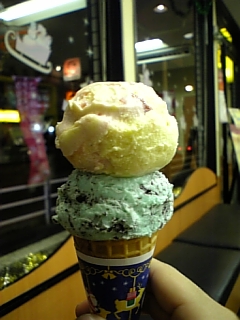In the photo, a hand holds a waffle cone with two scoops of ice cream, delicately stacked. The bottom scoop, light green in color, seems to be mint chocolate chip, while the top scoop, yellow and possibly caramel-infused vanilla, sits impressively above it. The cone itself is wrapped in blue and yellow paper, adorned with a design featuring a merry-go-round animal.

Behind the cone, the setting appears to be an ice cream shop. Large glass windows reflect the interior lights, and outside the shop, you can see a white rail. Inside, next to the windows, is a long wooden bench topped with black cushions, inviting patrons to sit and enjoy their treats. This detailed scene captures a moment of delightful indulgence in a cozy and inviting environment.